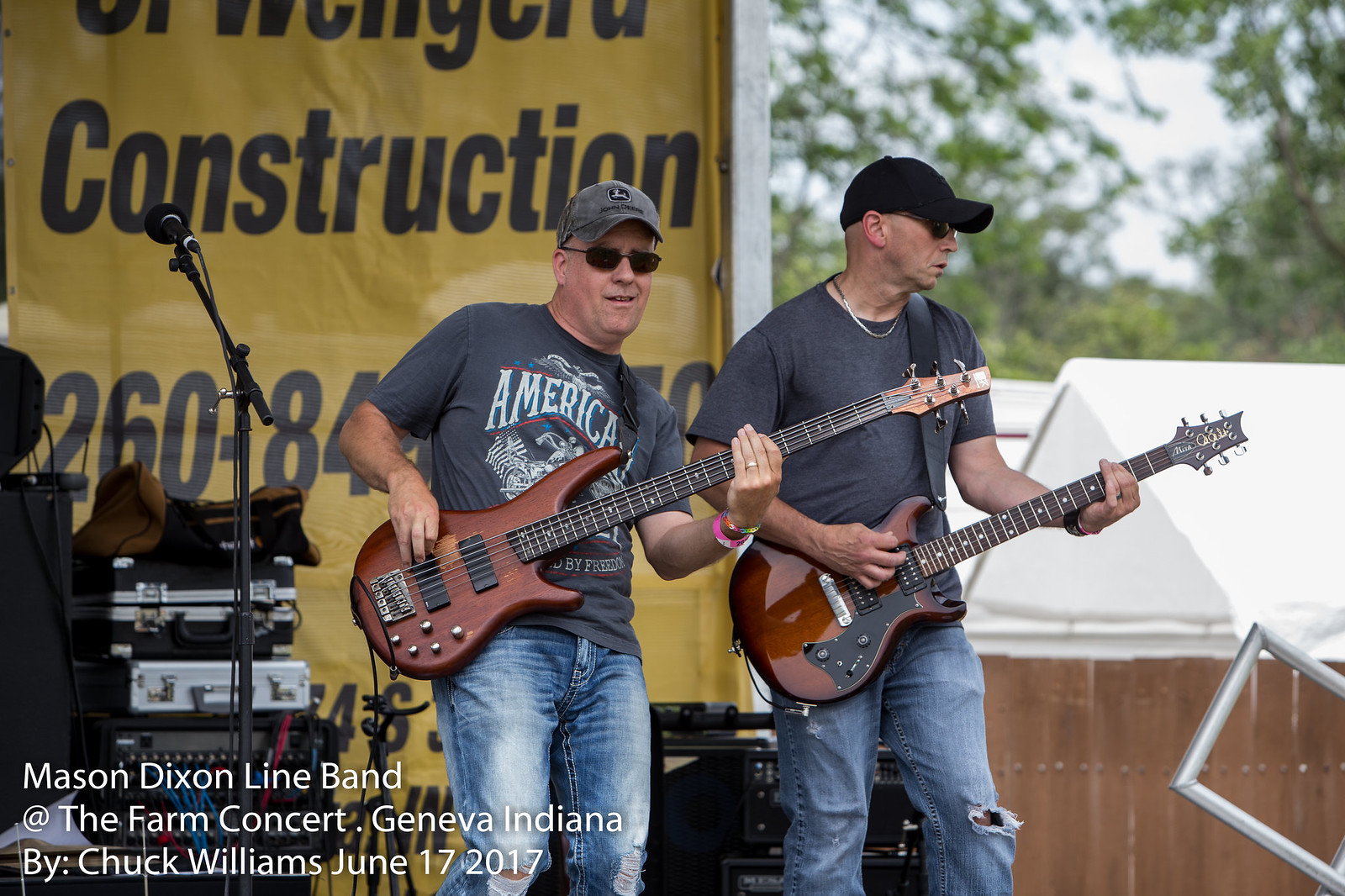The photograph captures two middle-aged Caucasian men performing on an outdoor stage during the day. Both are dressed in gray short-sleeved shirts and blue jeans, with baseball caps – the man on the left wearing a gray hat and the one on the right in a black hat. They both have black sunglasses on and are playing dark brown guitars. Their facial expressions and posture indicate they are actively engaged in their performance. 

To the left of the men, a microphone stand and various audio equipment, including amps, are visible. A prominent mustard yellow banner occupies the left side of the background, featuring black text that includes the word "construction" and a phone number, though these top words are not completely readable. 

Adding depth to the atmosphere, the overcast sky and leafy green trees are visible in the upper right corner of the image, emphasizing that the event is taking place outdoors. Additionally, some white tents and a fence can be seen behind the performers. The yellow banner also highlights the name "Mason Dixon Line Band," indicating the band's identity and possibly promoting the concert they are performing at.